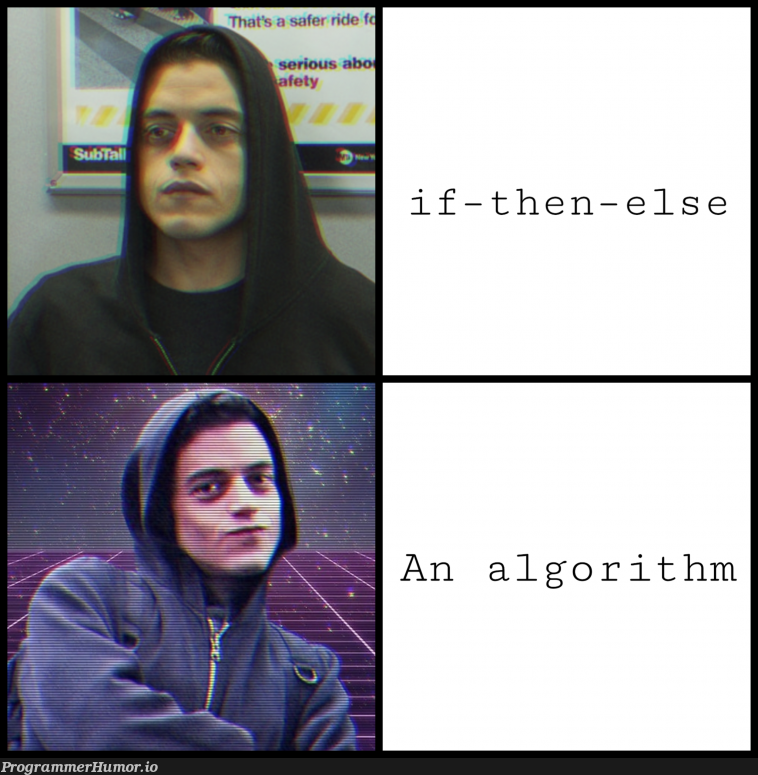The image is a programming humor meme, formatted as a large square with a black border, divided into four quadrants. The upper left quadrant features a young man, possibly named Pete, with brown hair. He's wearing a dark hoodie pulled over his head and is sitting in front of what looks like a poster, potentially unrelated to the content. The upper right quadrant contains the text "if - then - else" in lowercase letters against a white background. The lower left quadrant shows the same man, now smirking at the camera with his arms crossed, against a starry background with purple-outlined squares at his feet. The lower right quadrant displays the text "an algorithm." At the very bottom left of the image, outside the four quadrants, the website "programmerhumor.io" is mentioned. This meme humorously plays on programming conditional statements and is likely intended for a programming-savvy audience.